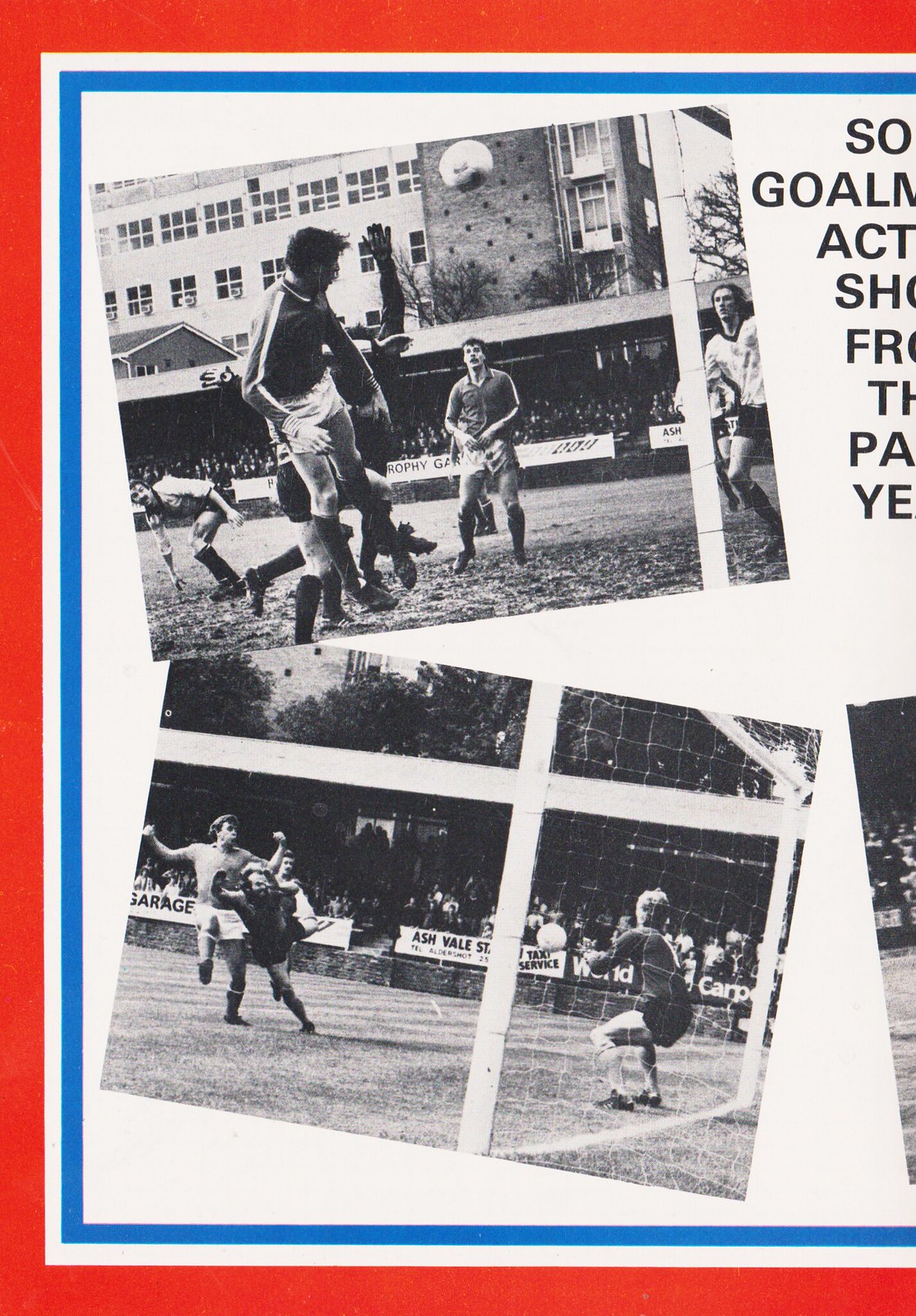This image appears to be part of a retro poster or program for a football club, and the right side is cut off. The visible portion features a red outer frame, a white inner frame, and a thin blue frame inside that. Centered within these borders, there are two black-and-white photographs of people playing football, seemingly in a stadium with fans visible in the background.

In the upper photograph, around three or four young men are captured mid-action, volleying for the ball. One player is notably in the air, heading the ball which is seen to the right, while other players look on, all standing on a grass field. Behind them is a three-story building, adding to the stadium ambiance. 

The lower photograph presents a different scene – a goalie is situated in front of a net, crouching and reaching out for a soccer ball that's nearing him. To his left, a player who likely kicked the ball is visible, as well as another player possibly attempting to block the shot. Together with these visual elements, there is a partial text in the top right-hand corner, but the fragmented lettering remains indecipherable.